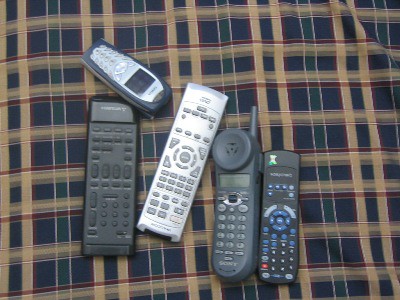This color photograph showcases an eclectic array of electronic devices resting on a dark brown and beige plaid fabric that could either be a tablecloth or a bedspread. The fabric features blue and green squares interspersed with red lines. The devices include five objects: three TV remote controls and two old-style cell phones.

Starting from the top corner, there's a nearly upside-down, outdated silver and black cell phone reminiscent of the late 1990s or early 2000s. Adjacent to this cell phone is an all-black remote control. Beside it lies another remote, this time silver with gray buttons. Next to this is a black cordless landline phone adorned with light gray buttons. The last item is a remote control characterized by its black body and distinctive blue-gray buttons, including a prominent red button. The devices are neatly arranged, providing a nostalgic glimpse into past electronic eras.